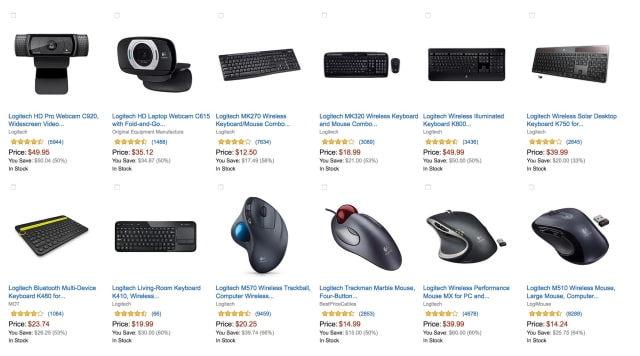The image background is white and lists various electronics in blue text. The text becomes blurry when zoomed in, making it challenging to read, but here is a structured attempt:

The top portion of the display seems to feature six items, as does the bottom portion, arranged as follows:

**Top Section:**
1. LongTek HD Pro Webcam, possibly C920 with widescreen video capabilities.
2. LongTek HD Laptop Webcam, maybe C615 with a foldable design.
3. LongTek MK270 Wireless Keyboard and Mouse Combo.
4. LongTek, model unclear, possibly MC320 Wireless Keyboard and Mouse.
5. LongTek Wireless Illuminated Keyboard K800.
6. LongTek Wireless Solar Desktop Keyboard K750.

**Bottom Section:**
1. LongTek Bluetooth Multi-Device Keyboard, possibly model K480 or K850.
2. LongTek Living Room Keyboard K410.
3. LongTek M570 Wireless Trackball Mouse.
4. LongTek Trackman Marble Mouse.
5. LongTek Wireless Performance Mouse MX, model possibly MX Master or MX Anywhere.
6. LongTek M510 Wireless Mouse.

Despite the blurriness, this appears to be a catalog of various computer peripherals by LongTek, including webcams, keyboards, and mice, with several models denoted by their respective features and designations.